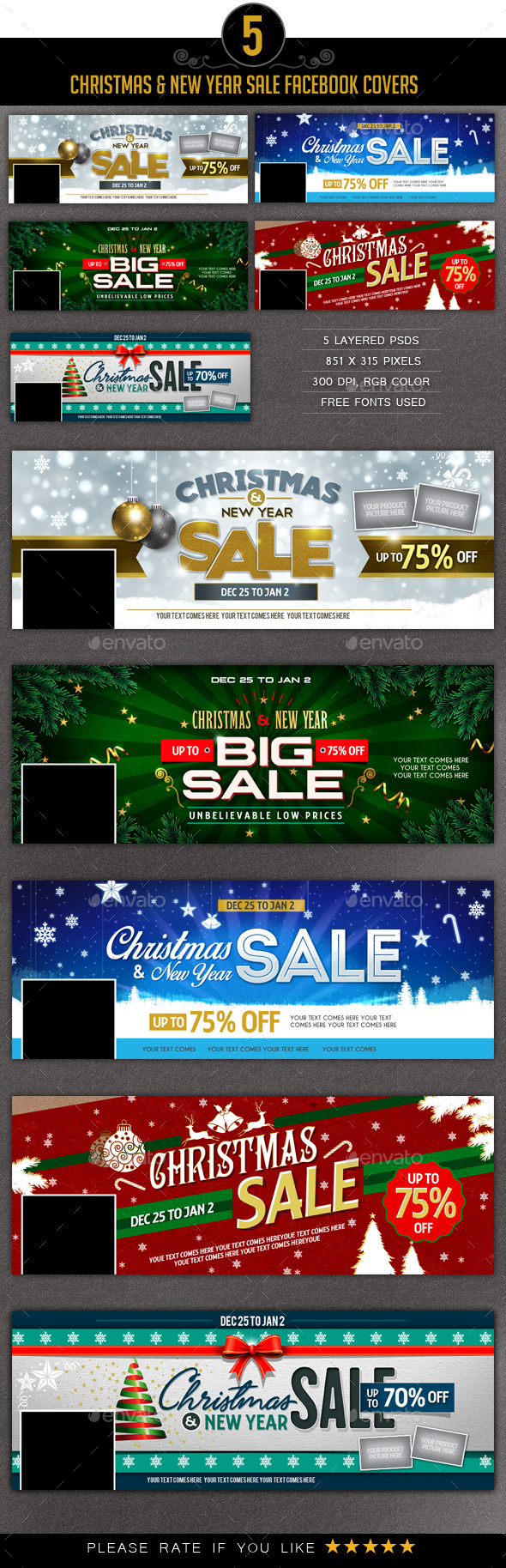The image is a screenshot from a phone displaying various sale advertisements. At the very top, centered in the screen, there is a bold number "5" inside a black oval background. Just below, a black rectangle contains the text "Christmas and New Year's Sale Facebook Covers." 

The display showcases multiple design options for sale covers, presumably for purchase and use on platforms like websites or Etsy stores. The designs feature a variety of backgrounds, colors, and fonts. Each design can be selected by clicking on it, and the options are labeled as "Five layered PSDs" along with their pixel dimensions. It also mentions that free fonts are used in these designs.

In total, there are ten different cover designs available. The top section contains smaller, condensed thumbnails of each design, while the bottom section enlarges these images, allowing for detailed examination. Each cover prominently displays text related to Christmas sales, such as discount percentages.

Additionally, there is a prompt at the bottom encouraging users to rate the designs, with a suggestion to give five stars if they are satisfied. Some of the designs at the top appear repeated in the larger images below for better visibility, emphasizing their festive Christmas theme and sale announcements.